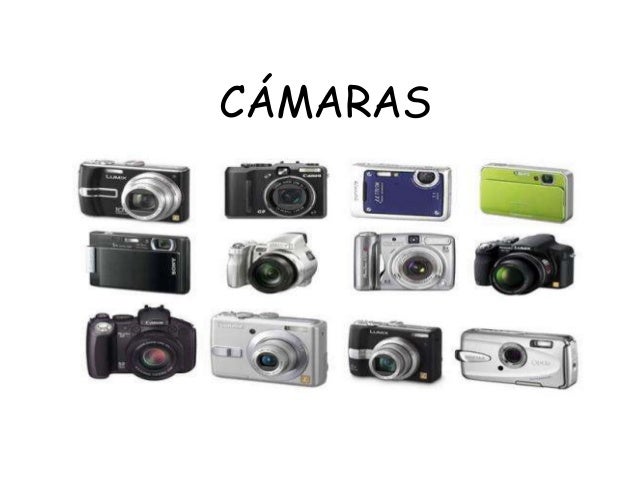The image depicts a collection of 12 modern, possibly digital cameras arranged in three rows with four cameras each on a plain white background. Above the cameras, the word "Cámaras" is written in a font resembling Comic Sans, suggesting it might be in Spanish. The top row features two black cameras on the left, followed by a blue camera and a green camera on the right. In the second row, there is a black camera, two silver cameras, and another black camera. The bottom row alternates between black and silver cameras. Some cameras have accents of color around certain areas like the lens, with at least four cameras having noticeably large lenses. The design of the cameras varies; some are boxy while others are flat, but they generally appear to be compact instant cameras.